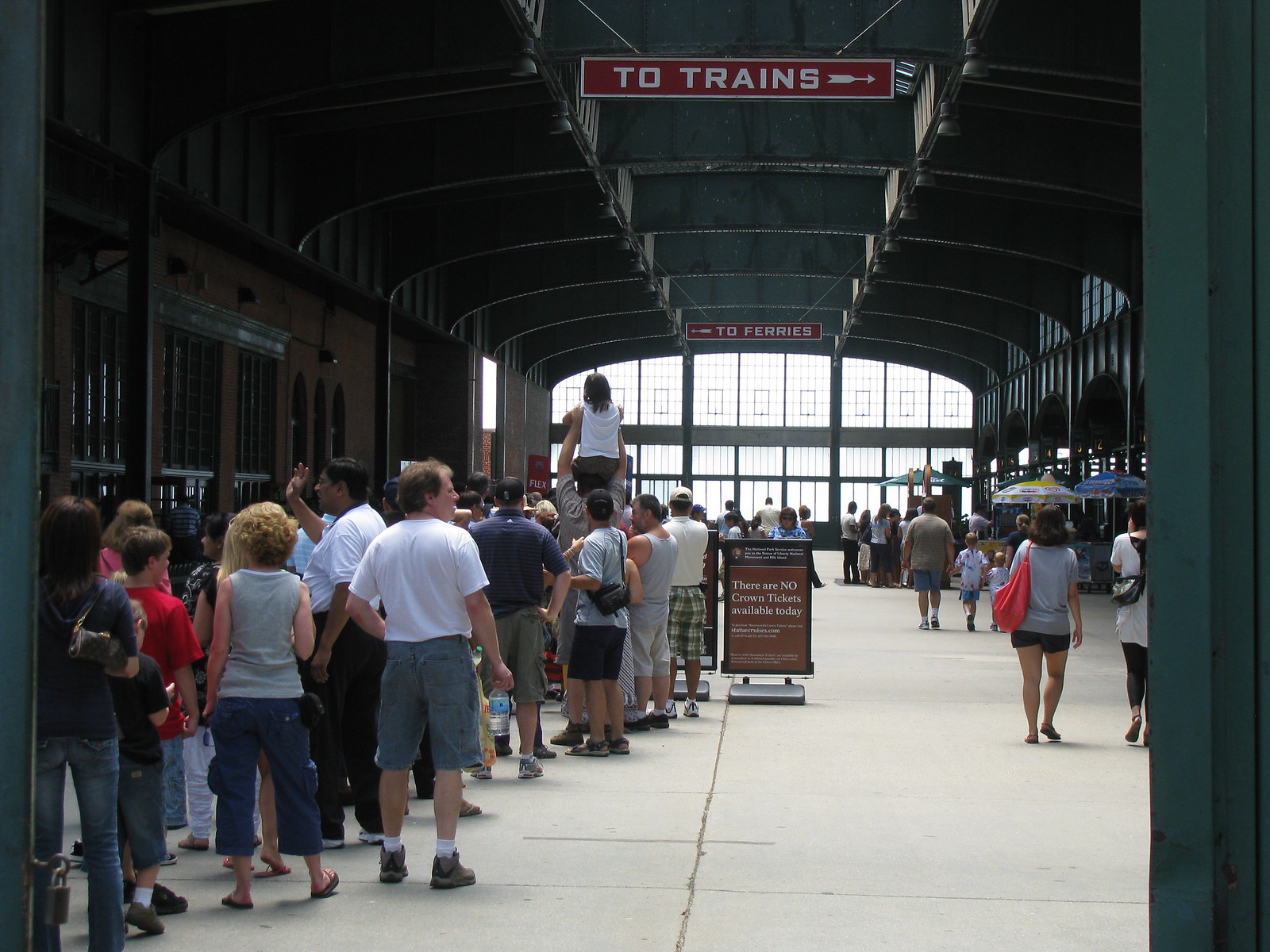The photograph captures the bustling interior of a large enclosed train station, featuring a significant number of people engaged in various activities. At the back of the image, a prominent expanse of large paned windows allows a flood of natural light, though the outside appears featureless and white. The station floor is composed of cement, bordered by walls on either side.

Hanging from the ceiling, two red rectangular signs provide directional guidance. The first sign, closer to the foreground, reads "To Trains" in white all-caps text with an arrow pointing to the right. This sign directs passengers towards the train platforms. Further back, another similar sign indicates "To Ferries" with an arrow pointing to the left, guiding travelers towards the ferry docks.

On the left side of the station, a long line of people stretches from the "To Ferries" sign towards the camera, composed of families, children, and adults casually dressed in blue jeans, shorts, tennis shoes, and the like. The most noticeable individual in the queue is a man carrying a child on his shoulders, who towers above the crowd. On the right side, various individuals walk towards the large windows. Among them, a woman carrying a red bag over her shoulder, dressed in black shorts and a blue t-shirt, is heading towards some seating visible in the distance, which includes cafe-style tables and umbrellas. Additionally, a man with two children holding hands moves away from the camera.

The station also features further details: On the left side near the wall, there appear to be windows likely for ticketing, set into a brick wall, adding a functional and architectural element to the bustling environment.